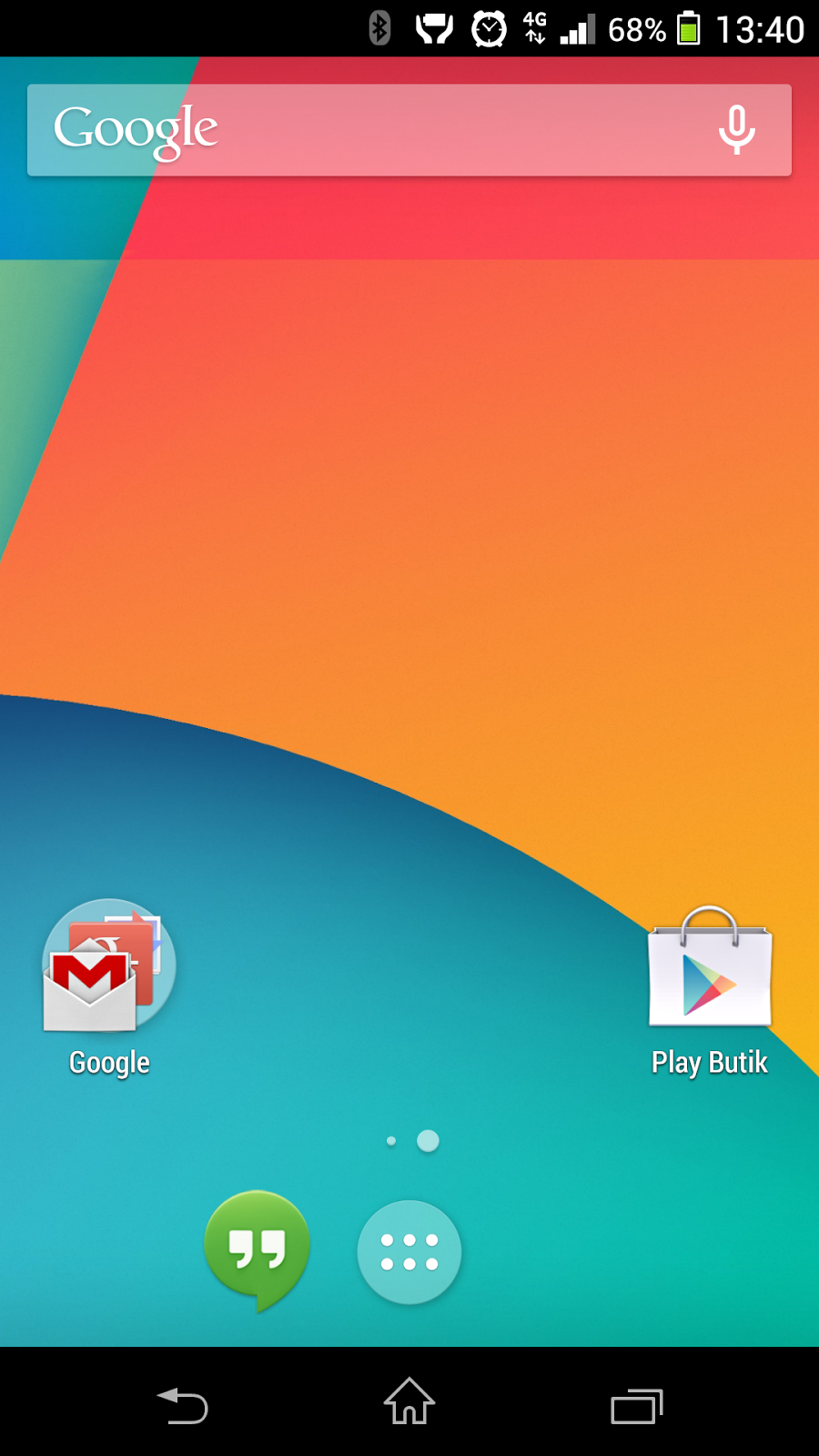A detailed screenshot of an Android smartphone home screen is presented. In the top left corner, the presence of the Google logo signifies that it is an Android device. The time is displayed in a 24-hour format, showing 13:40, and other indicators in the top right include a battery life at 68%, a 4G network connection with three bars of signal strength, an alarm clock icon, and a dim Bluetooth symbol indicating it is turned off.

Prominently located at the top of the home screen is the Google search bar. The wallpaper features a vibrant, multi-color design with shades of blue, green, yellow, and red. Below the wallpaper, there are several app icons including Google, the Play Store, and a messaging app. At the very bottom of the screen, navigation buttons are clearly visible: the back key on the left, the home key in the center, and the options key on the right. Notably, the overall design and layout suggest this is an older version of the Android operating system.